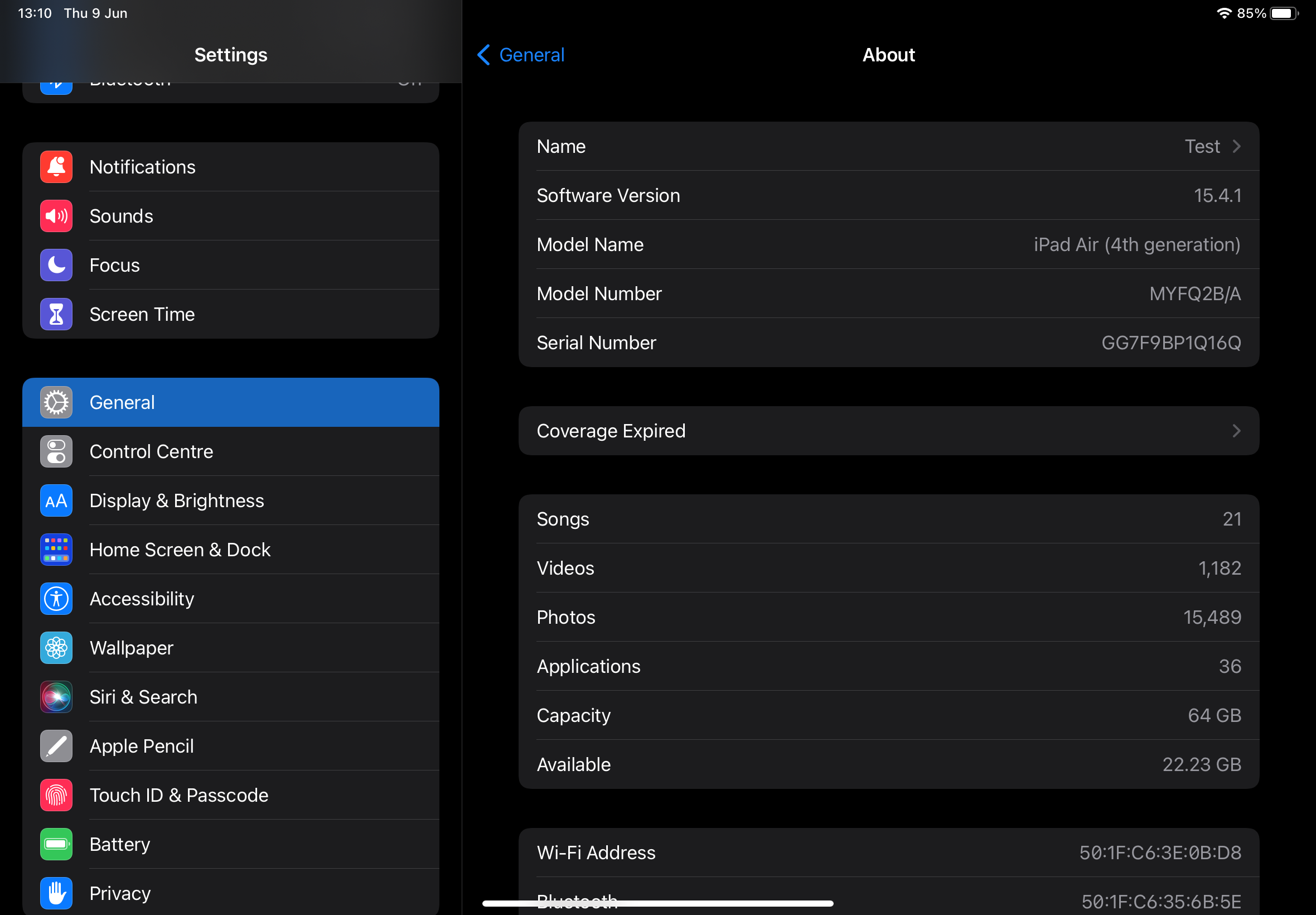This is a detailed screenshot of an Apple iPad, specifically an iPad Air 4th Generation, displayed in landscape mode. The image reveals the device's "Settings" menu, focused on the "About" page within the "General" section. The iPad's name is listed as "test," and it runs on software version 15.4.1. The screen indicates that the device’s coverage has expired. In terms of media and storage, the iPad contains 21 songs, 1,182 videos, and 15,489 photos, with 36 applications installed. The iPad has a capacity of 64 gigabytes, of which 22.23 gigabytes are available. Additional details such as the model number, serial number, Wi-Fi address, and Bluetooth address are also visible. The settings interface is in dark mode, presenting a black or dark gray background with white or light gray text. On the left-hand side of the screen, a list of other settings options, such as Control Center, Display & Brightness, and Home Screen, can be seen.